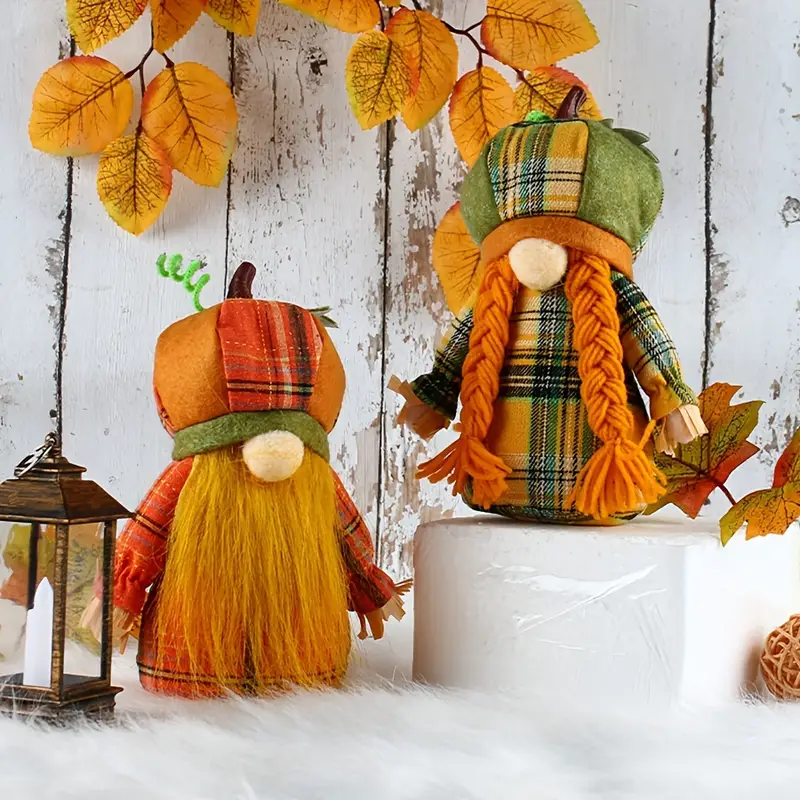In this detailed and whimsical photograph, we see two charming stuffed gnome dolls dressed in tartan-patterned garments evocative of autumnal and Scottish themes. Both gnomes don beanie-like hats adorned with pumpkin stem tops, covering their faces except for their round, tan noses. The first gnome, positioned on the right atop a white, blocky platform, wears a green, orange, yellow, and black tartan robe. This gnome features two long, orange braids made of yarn. The second gnome, situated on the left, is cloaked in a red, yellow, and black tartan and sports a long, orange beard, enhancing its male characterization. Their hands appear to be made of straw, further adding to their rustic charm.

The backdrop is a weathered white wood wall with patches of paint missing, lending a vintage feel to the scene. Above, orange and yellow leaves mingle with brown stems, enhancing the autumn atmosphere. To the left of the gnome dolls stands a brown lantern with a visible candle inside, adding a cozy touch. The floor is covered with a wispy, shaggy white cloth or carpet, complementing the overall setting.

Overall, the image captures a quaint, seasonal vibe, marrying elements of fall and traditional Scottish attire in a delightful gnome-themed display.